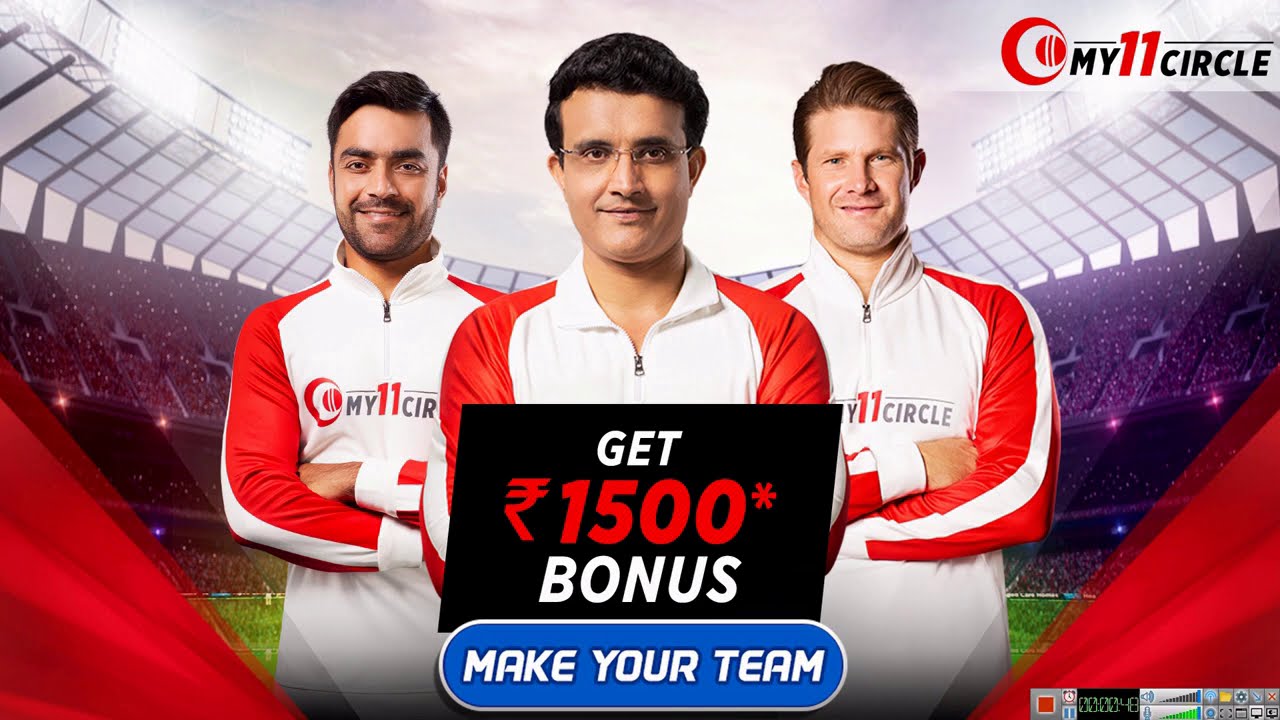The image is a screenshot taken from a TV or computer monitor, depicting three men standing in a soccer stadium. The men are arranged in a triangular formation, with one in front and two behind him on either side, all facing the camera with their arms crossed and smiles on their faces. They are wearing identical white and red striped racing jackets, reminiscent of sports jerseys. The man in the front has dark hair and eyeglasses, while the man to his left has dark hair, a dark mustache, and a dark beard. The man on the right has red hair. 

In the background, there is a graphical design mimicking a soccer stadium, complete with visible seats and grass. Superimposed in front of the men, there is a black parallelogram with three lines of text: "GET ₹1500 BONUS" in white and red letters, and beneath it, the line "MAKE YOUR TEAM" in white letters on a blue background. In the upper right-hand corner, there is a logo consisting of two concentric circles in red, surrounding the text "My 11 Circle," with "11" highlighted in red.